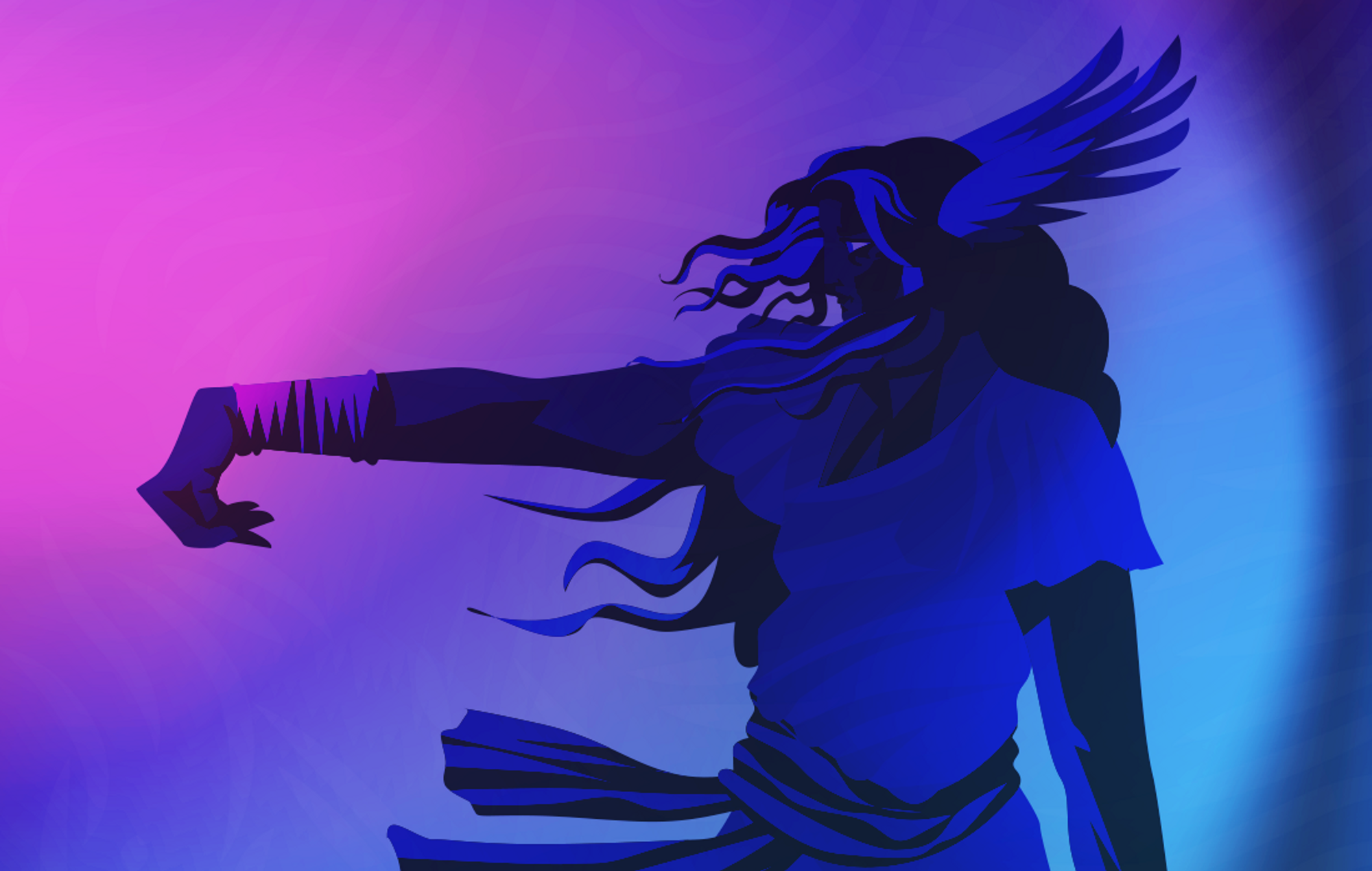This image portrays an animated character combining both human and animalistic traits, set against a vibrant, color-gradient background. The figure, which might evoke Native American aesthetics, has long, dark hair flowing dynamically, accompanied by sections of light blue or white strands that create a striking contrast. Notably, the person's head features wing-like structures resembling bird wings, positioned where their ears would be.

The character stands with their right arm outstretched, the hand bent down and fingers pointing back toward them, adorned with some accessory on the wrist. Their other arm rests by their side. Clothed in a short-sleeve, light-colored shirt, the character has sashes around their waist with black stripes, fluttering in the wind toward the left.

The image itself is framed within a horizontal rectangle. The background transitions from light purple in the upper left to a richer blue on the right, with the bottom right corner deepening into a darker blue. The character's powerful, intent gaze is directed leftward, where the interplay of colors seems to produce a soft, illuminating effect. This expressive visual is either a colored drawing or a CGI creation, merging artistic elements harmoniously.